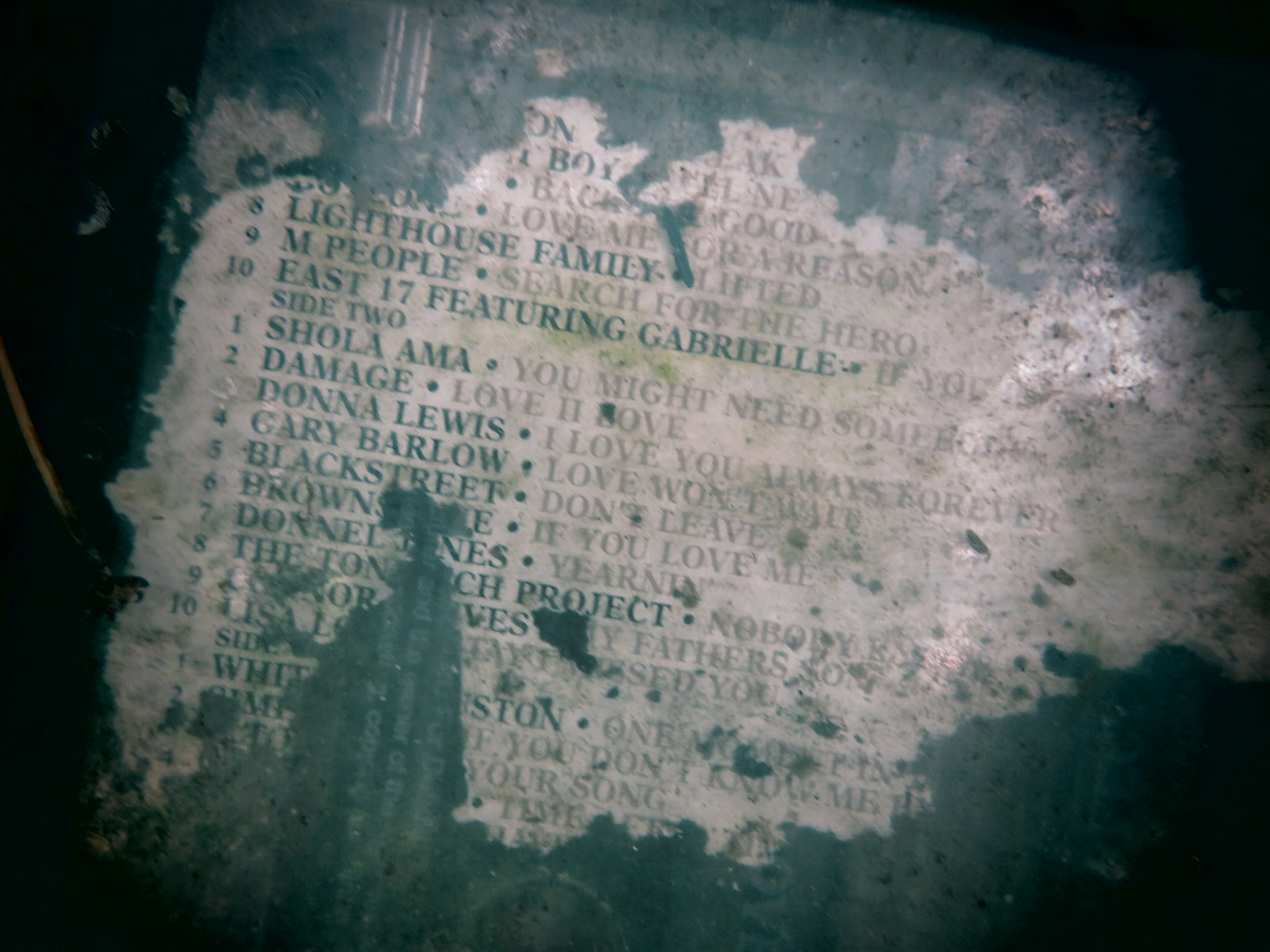This image features a single worn object positioned centrally against a dark background, possibly situated in a dimly lit room or outdoors at night. The object appears to be an old, bluish stone with faded, pale white text and symbols, as well as segments of torn paper that seem as if they've been peeled off like wallpaper. The paper, which has a whitish hue with gray and dark blue lettering, contains a list of song titles and artists' names. The text includes "Lighthouse Family" with the number 8 next to it, "M People - Search for the Hero" at 9, and "East 17 featuring Gabrielle" at 10. Another part of the list shows "Shola Ama" at 1, "Damage" at 2, "Donna Lewis" at 3, "Gary Barlow" at 4, and "Blackstreet" at 5. The object is quite weathered and dirty, suggesting its original white or tan surface has deteriorated, covered in patches of green or black grime. The rest of the text is largely illegible due to the worn and dirty condition of the object.